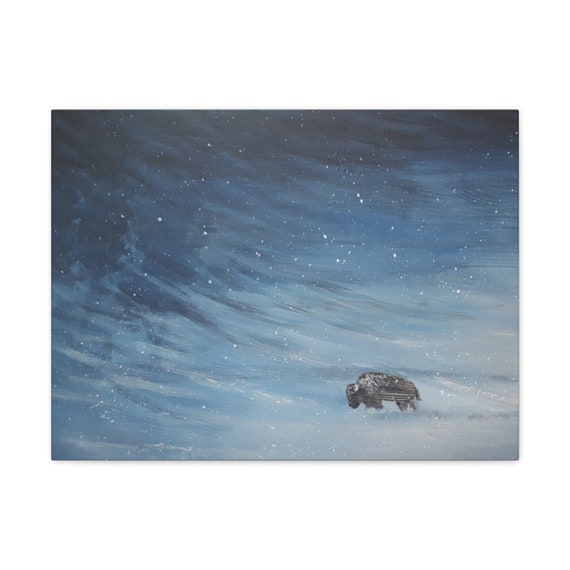The image is a detailed painting of a dark grey car and a bison enduring a fierce snowstorm in a snowy landscape. The painting, landscape-oriented and almost square, features a dark grey car near the bottom right, partially covered by accumulated snow. The whole scene is dominated by the storm, which transitions from lighter blues and greys in the bottom right to darker shades towards the top left, with the snow falling heavily in the form of white dots. 

Amidst this tumultuous weather, a bison struggles forward in the bottom right quadrant. The bison, depicted in profile with its head facing left and its tail to the right, has snow accumulating on its back, emphasizing the intensity of the conditions. The storm's movement appears to sweep from the bottom right to the top left, contributing to the dramatic atmosphere of the piece. The painting evokes a sense of resilience and perseverance, as both the car and the bison continue through the storm, aiming to find safety amidst the harsh, wintry environment.